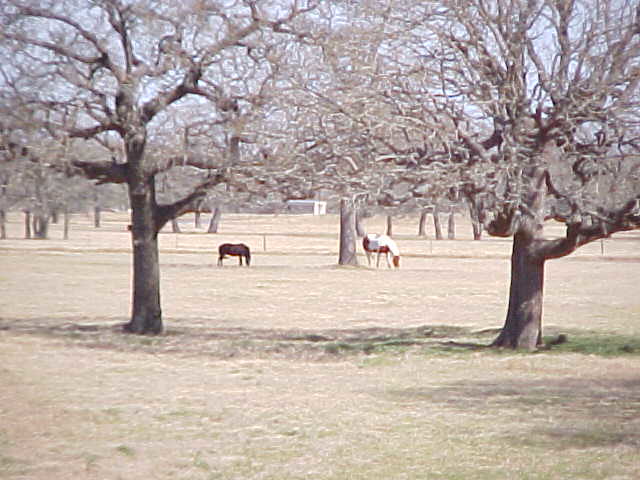A serene photograph captures an expansive field during late autumn. The scene features a mix of pale green and straw-colored grass, hinting at the season's chill. Just right of center, a white horse speckled with brown grazes peacefully with its head down, while to the left of center, a black horse mirrors this behavior. Both horses are intent on their meal in an otherwise quiet landscape. Surrounding them, a sparse collection of leafless trees extends their barren branches skyward; these trees could be oaks or apple trees, stripped of their foliage by the cold. The gray, overcast sky looms above, adding a touch of melancholy to the scene. In the far distance, barely visible through the trees, a building stands, subtly hinting at human presence in this tranquil countryside setting.